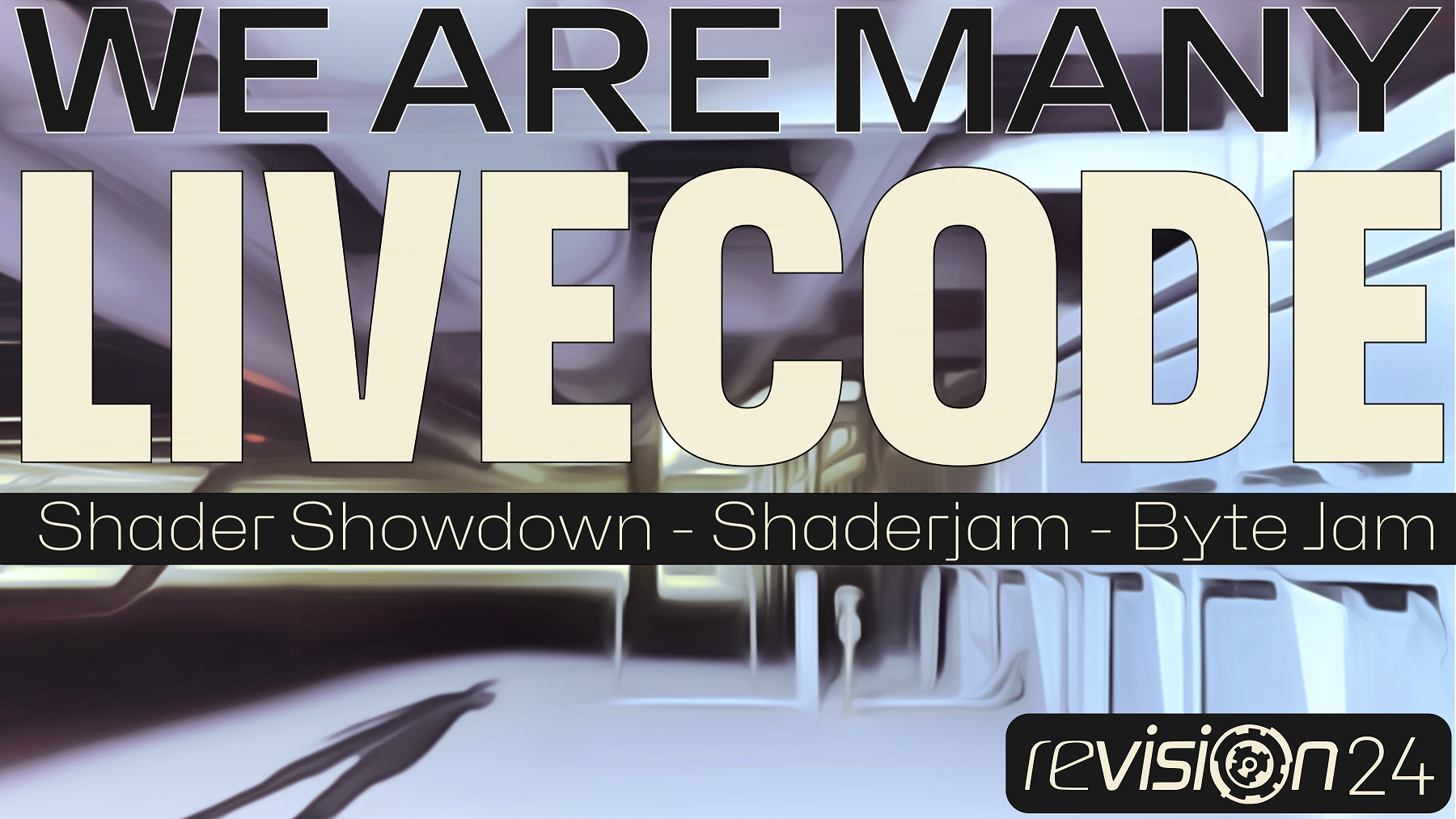This digital image advertisement depicts a futuristic, underground train station-like interior environment. The space features white walls, a long hallway with light streaming in from the left, and a light blue ground with some framin on the right side. Shadows of two people are visible in the bottom left corner, adding depth and intrigue to the scene.

Overlaid on the image, though rather than exclusive to the top, are three central lines of text spanning the entire width of the image. The first line, "We are many," is in prominent black text with a white outline. The second line, "live code" written as a single word, appears just below in a light tan or beige color. The third line is enclosed in a black rectangle featuring, in white text, "Shader Showdown/Shader Jam/Byte Jam" (with Byte spelled B-Y-T-E).

In the bottom right corner, set within another black rectangle with curved corners, is the brand name "Revision 24," rendered in the same light tan color as the second line of text. This detailed composition combines modern typography with a high-tech environment to create a compelling visual statement.